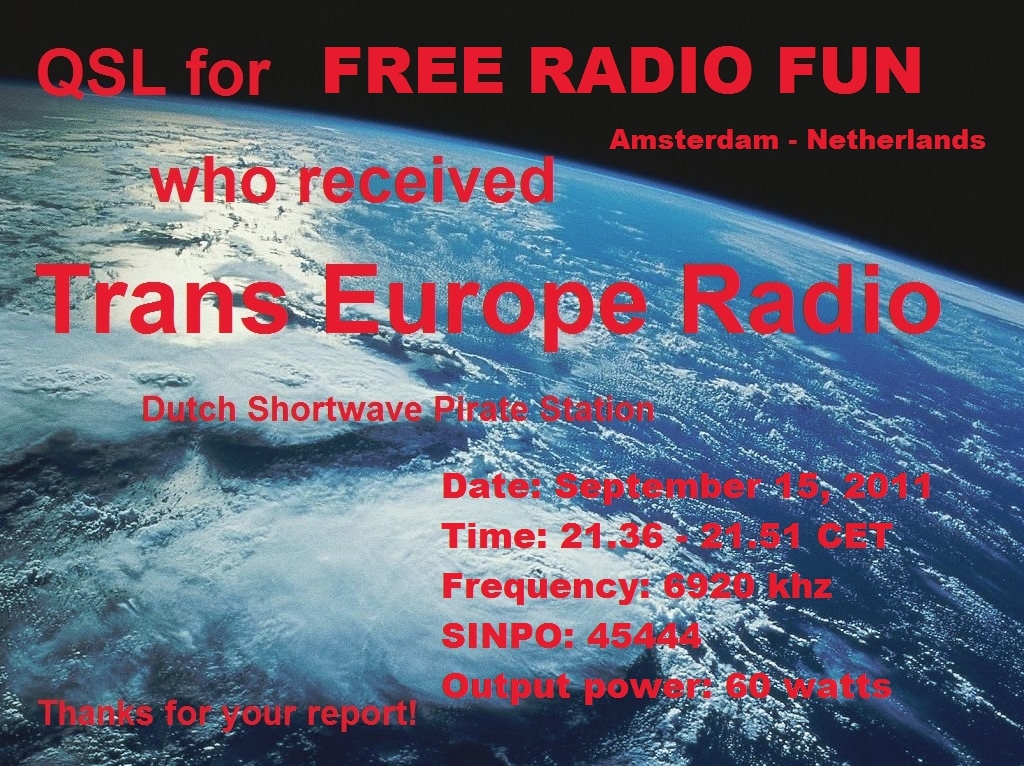The image is an advertisement for a radio event or station titled "QSL for Free Radio Fun" in Amsterdam, Netherlands, organized by Trans Europe Radio, a Dutch shortwave pirate station. The background prominently features a photograph of the Earth as seen from space, showcasing a vast expanse of blue ocean with white specks and thick cloud formations, especially noticeable at the bottom center. The surrounding area outside of the Earth is pitch black, emphasizing the planet's curvature against the cosmos. Vibrant red text covers the image, detailing the event information: the date is September 15th, 2011, the time is 9:36 to 9:51 p.m. CET, and the frequency is 6920 kHz. Additional technical specifics include a SINPO code of 45444 and an output power of 60 watts. A small note in the bottom left corner expresses gratitude for audience reports.